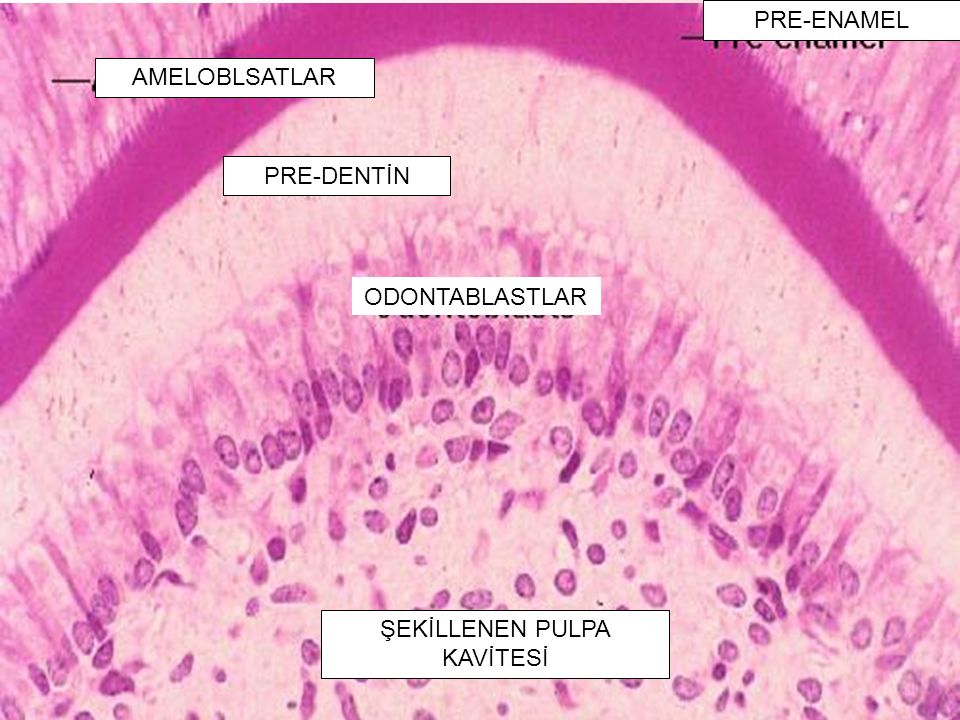This highly detailed, zoomed-in photograph depicts various layers of a developing tooth, emphasizing the complex stages before enamel formation. The image is rendered in a palette of pinks, reds, whites, and occasional purples, with each layer clearly demarcated by color and labeled in black text. In the upper right corner, the label "pre-enamel" can be seen. The topmost layer features reddish-pink lines labeled "amylobalsatlar". Below, there is a distinct pink ring labeled "pre-enamel". Moving downward, a lighter pink ring is marked "predentin", followed by a bubbly, popcorn-like ring labeled "odontoblastlar". The bottom section, dotted with numerous small purple elements, contains the label "cichlonin pulpocavities". While these terms appear to be in a foreign language, their context suggests a scientific explanation of the dental development process, possibly an educational resource for understanding how a tooth forms before the enamel layer is completed.